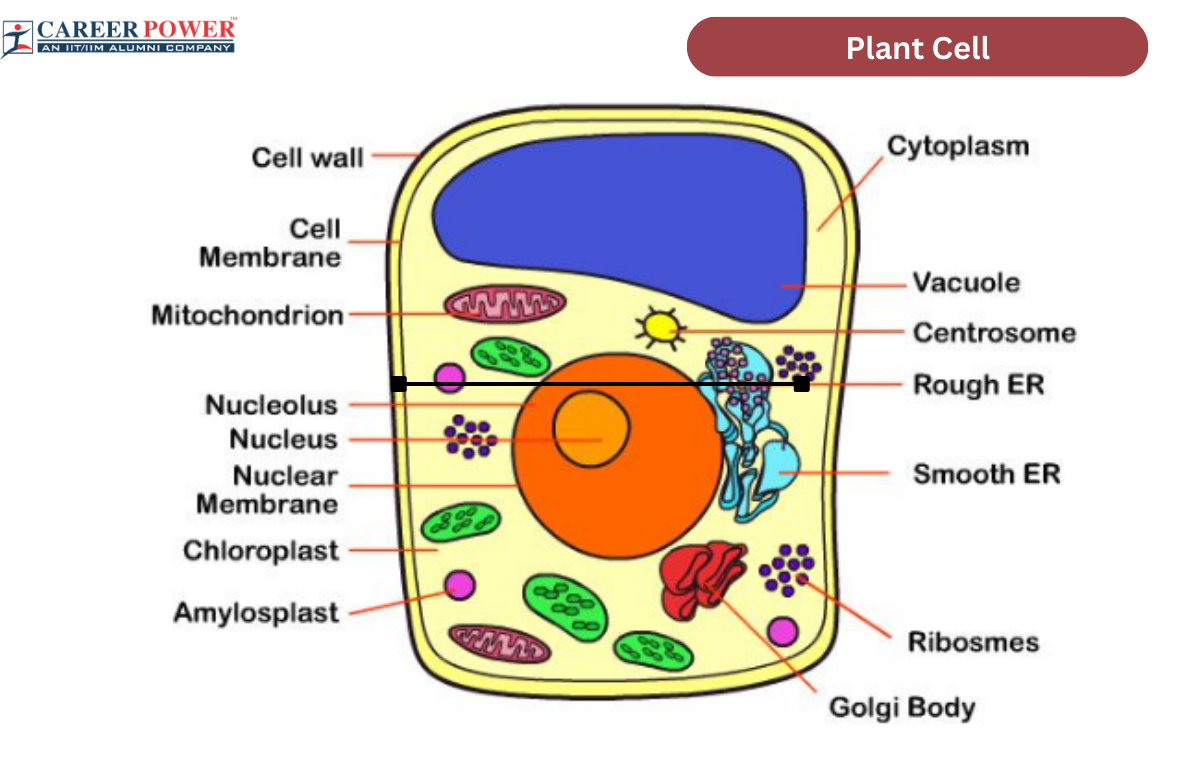The image is a detailed diagram depicting a plant cell, characterized by its elongated, round-edged rectangular shape. The label "Plant Cell" is prominently displayed in white font on the upper right-hand corner of the image.

The central focus of the diagram is a squarish, elongated, yellow structure, representing the plant cell itself. Within this structure, several key components are illustrated and labeled. The upper section of the cell is highlighted in blue, possibly indicating a specific organelle or cell region. Centrally located within this area is a prominent, round orange circle with a lighter orange circle situated almost to the left of its center, symbolizing the cell nucleus and its nucleolus.

Additional circular elements are dispersed throughout the cell's interior, each linked to detailed labels on both the left and right sides of the diagram. These labels, connected by precise lines, identify various critical organelles and structures within the plant cell, providing a comprehensive understanding of its intricacies.